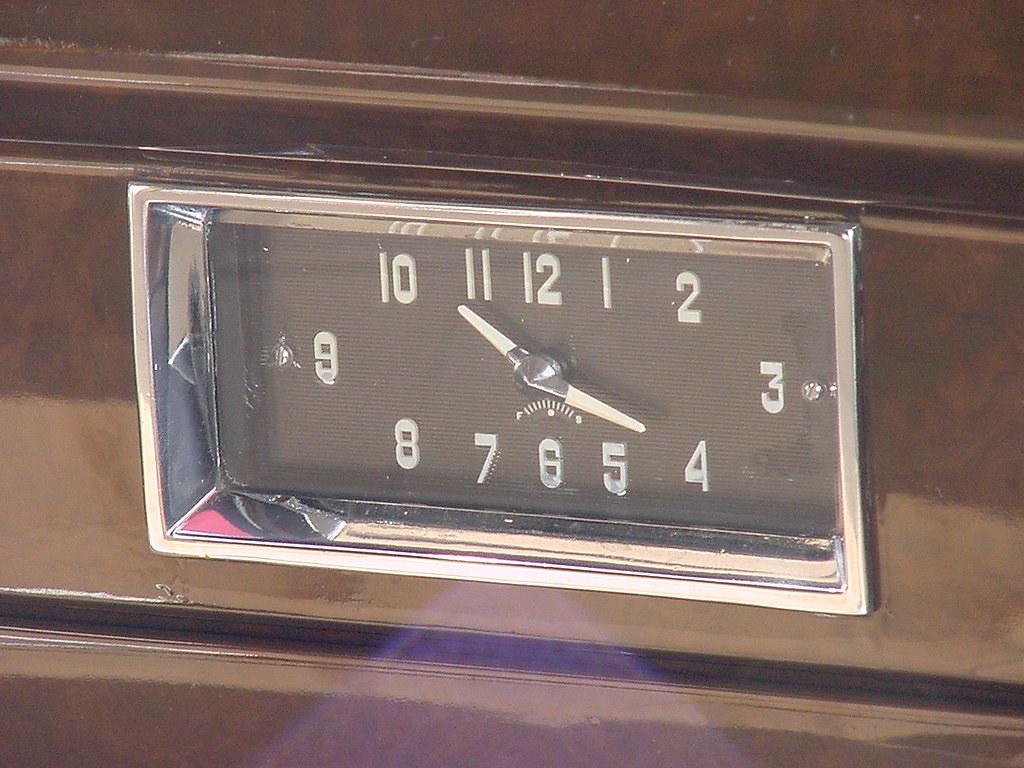The image features a close-up shot of an antique clock, rendered in exquisite detail. The clock is encapsulated in a shiny brown, square or rectangular frame with a silver outline, evoking a sense of timeless elegance. Its face is predominantly black, accentuating the stark white hands and numerals. The numerals appear as though they’ve been manually inserted, reminiscent of the style from about 50 years ago, giving the impression of hand-crafted authenticity with a slightly irregular placement. Centrally, the clock sports a black core, further contrasting the white, slender hands. Below the clock hands, an additional feature is visible, resembling an alarm-setting mechanism, adding to the clock’s functional charm and vintage allure.